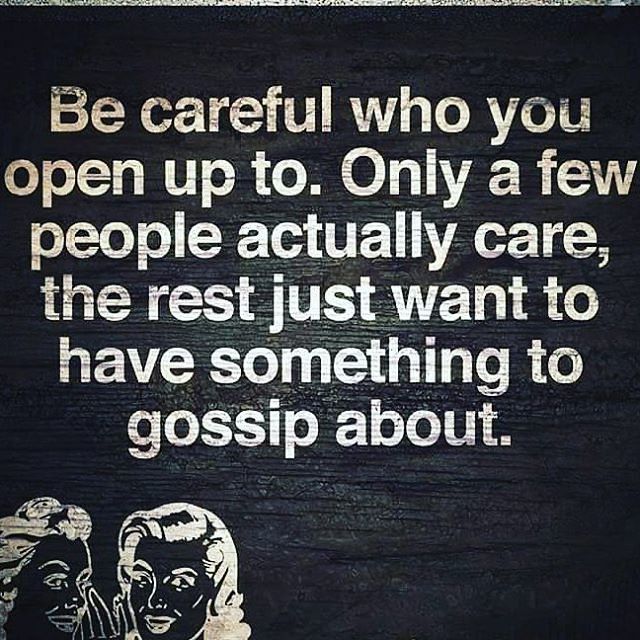The image presents a vintage or retro-style illustration with a rustic aesthetic, featuring a dark, textured background that resembles aged wood. Centered in white, distressed lettering, the text reads: "Be careful who you open up to. Only a few people actually care; the rest just want to have something to gossip about." This text dominates the upper portion of the image and appears to have the background texture visible through it, adding to the worn, aged look. In the bottom right corner, two human figures—depicted as women with clear facial features and retro-style curly hair—are engaged in a conversation. One woman is holding her hand up, seemingly whispering to the other. The overall design, with its contrasting white elements against a dark backdrop and detailed character illustrations, suggests a relatable piece that could be displayed as a decorative sign in a home or business.